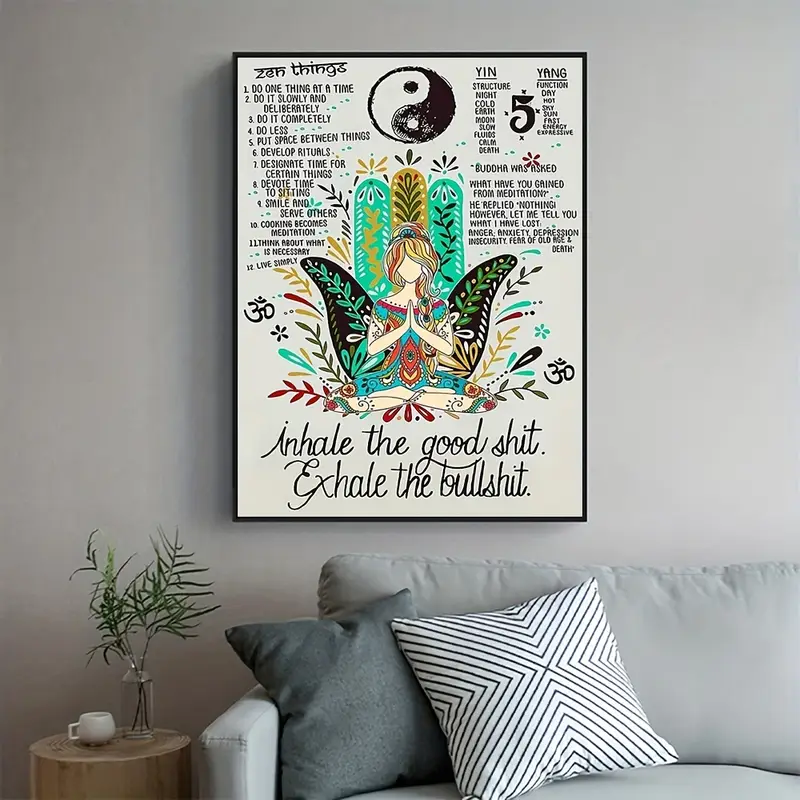In the photograph, a cozy section of a living room is depicted with a focal point on an eye-catching motivational poster hanging on a gray wall. The poster, encased in a black frame and measuring approximately 30 by 36 inches, is rich with details. Dominating the poster is a colorful illustration of a Hindu hand symbol painted in green, yellow, and black. Seated in front of this vibrant hand is a meditative woman with long blonde and red hair, adorned with a tiara. She wears a pink, blue, and red outfit and has what appear to be ankle bracelets or tattoos. Her hands are brought together at heart center in a classic yoga pose, with her legs crossed in a lotus position. Above her, a yin-yang symbol in black and white introduces the poster, which is further adorned with elements that emphasize balance and mindfulness.

The text around the central image accentuates the theme of Zen living. At the top, the heading says "Zen Things," followed by numbered items like "Do one thing at a time" and "Do it slowly and deliberately." The list includes suggestions for cultivating a calm and focused lifestyle. Towards the bottom, the poster boldly states, "Inhale the good shit, exhale the bullshit," adding a touch of humor.

The living room itself features a gray couch with two pillows: a darker gray pillow and another with a black-and-white geometric diamond pattern. To the side of the couch is an end table that holds a small coffee cup and a glass vase with a green leafy plant, contributing to the room’s serene ambiance. The overall atmosphere blends minimalistic decor with an inspirational touch, creating a welcoming space that exudes tranquility and motivation.